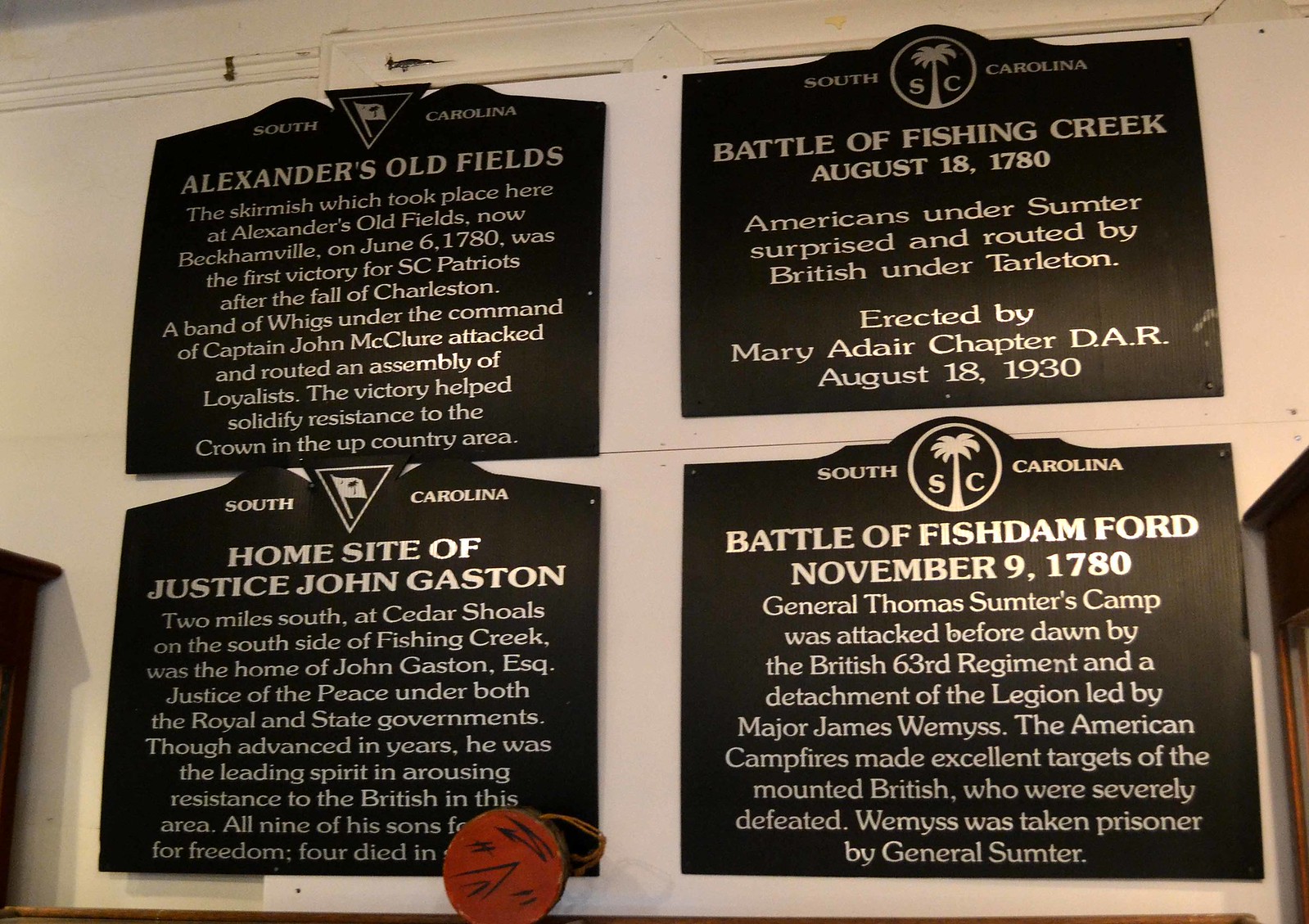The image shows a pristine white wall adorned with four black plaques that feature silver writing, each dedicated to significant historical sites and events in South Carolina. The plaques are uniformly styled with a "South Carolina" heading accompanied by a logo featuring a palm tree and the letters "S" and "C."

In the top-left corner, the plaque titled "Alessandra's Old Fields" briefly details a historical scheme that took place in this location. Directly to its right, another plaque titled "Battle of Fishing Creek, August 1780" recounts how American forces under Sumter were surprised and defeated by British troops under Tarleton, credited to the Mary Adair Chapter, DAR.

On the bottom-left, the plaque titled "Home Site of Justice John Gaston" notes that two miles south at Cedar Source on the south side of Fishing Creek was the residence of John Gaston. Adjacent to this, in the bottom right, the plaque labeled "Battle of Fish Dam Fork, November 1780" provides a summary of this pivotal encounter.

Additionally, below all these plaques, there is a notable red circular artifact, marked with various scratches, suggesting previous interactions or annotations by visitors.